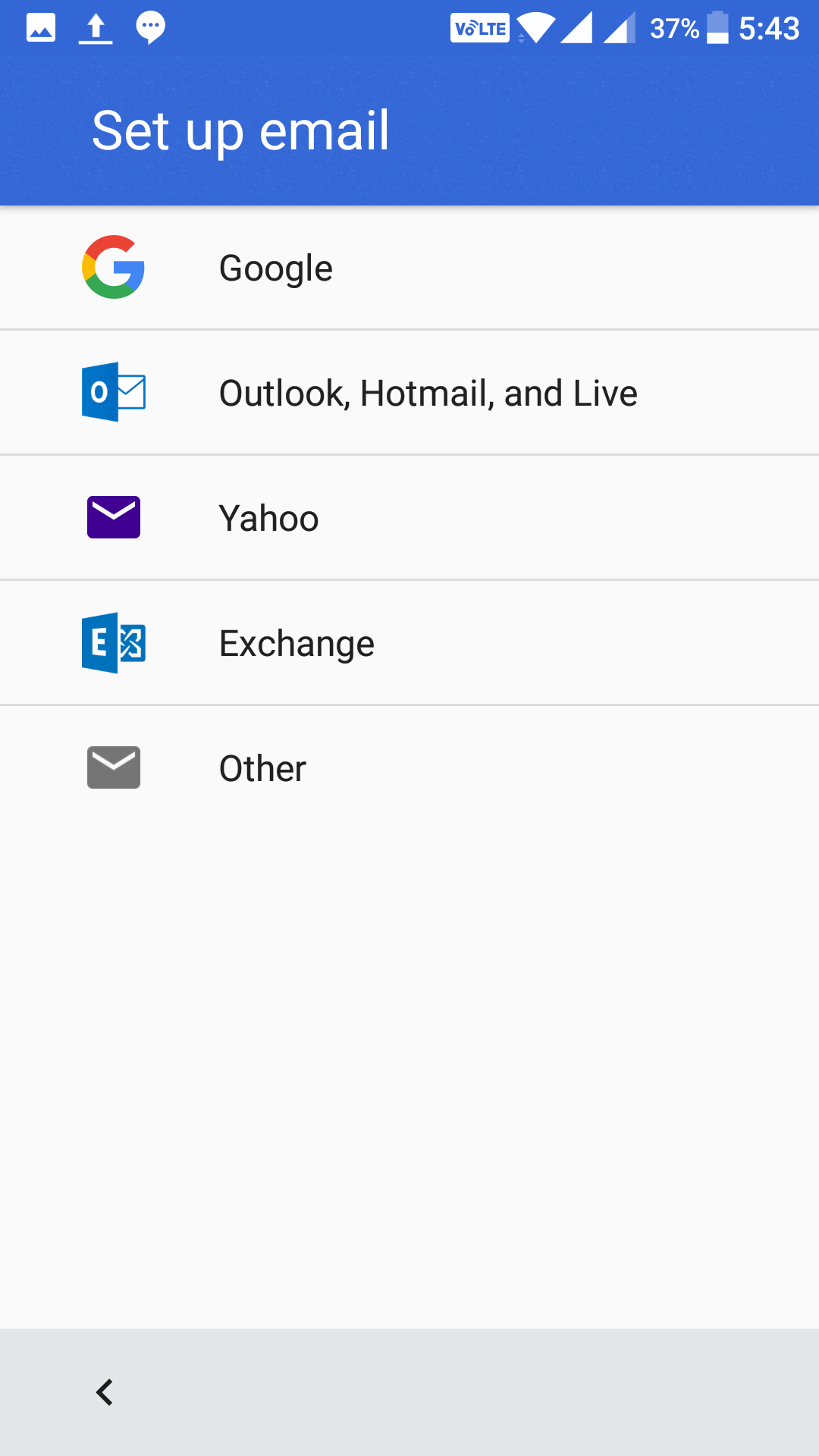The image, captured from an iPhone, shows the phone's status bar at the top, indicating it is 5:43 PM with a battery level at 37%. It has full network signal strength and displays "V-Lite LTE," signifying it is not connected to Wi-Fi. On the left, icons for download, a speech bubble with three dots, and a square are visible.

Below the status bar, a blue navigation bar reads "Set up email." The main content displays various email service options starting with "Google," represented by its multicolored 'G' logo. Following that is "Outlook, Hotmail, and Live," indicated by a white envelope icon partially enclosed by a blue square featuring a white 'O.' Next, "Yahoo" is shown with its distinctive purple envelope logo. Further down, "Exchange" is represented by an 'E' on an open blue square, revealing another square with a design. At the bottom, a generic grey envelope icon represents the "Other" email setup option.